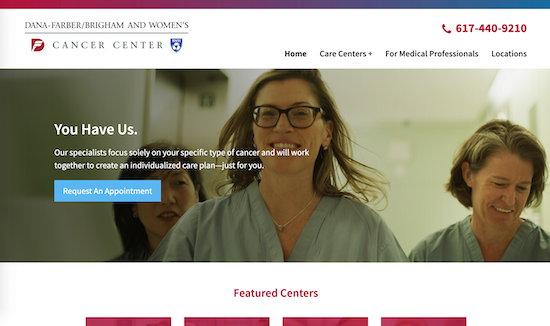The website appears to be for the Dana-Farber/Brigham and Women's Cancer Center. The header displays the center's name along with two emblems – one red and one blue. To the right, a red phone number is listed as 617-440-9210. Below the header, navigation links include "Home," "Care Centers," "For Medical Professionals," and "Locations."

The main image features a woman with glasses, smiling broadly, flanked by female doctors and nurses. The doctor on her right (our left) is an Asian woman, while the one on the left (our right) is an older white woman with some gray hair visible. All three women are dressed in teal or light blue uniforms, suggesting they may be nurses or medical staff. The background of the image includes an elevator and a corridor, with a light fixture in the upper right corner.

Beneath the image, the heading "Featured Centers" is displayed in red, followed by four rectangular red buttons. The specific content of these buttons is not mentioned, but they likely direct users to different sections of the website. The older white woman appears to be looking down at something, perhaps amused by a comment, while the main woman in front has a slight smirk on her face. This image and the website offer contact information and navigation options for accessing various cancer care services.